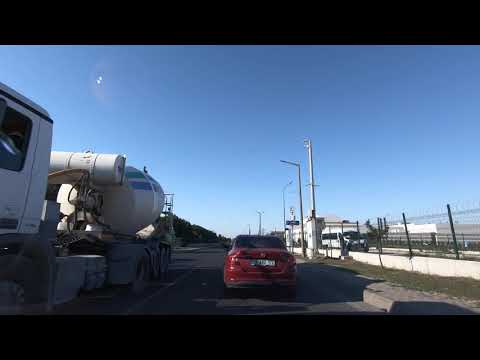Under a bright, clear blue sky, a red sedan is prominently captured traveling away from the viewer, likely photographed from a dash cam of the car behind it, on a multi-lane road. To the left, a large white truck, identified as a cement truck with its mixer visible, is heading in the opposite direction. The right side of the road features a black metal fence, potentially a chain-link with barbed wire, surrounding an industrial site or factory characterized by white buildings partly obscured in the distance. The scene also includes some greenery and light poles along the fenced area. The sidewalk, primarily gray with some stones, lines the road. Shadows of the red sedan and the white truck stretch across the road, suggesting it is midday with the sun high in the sky.